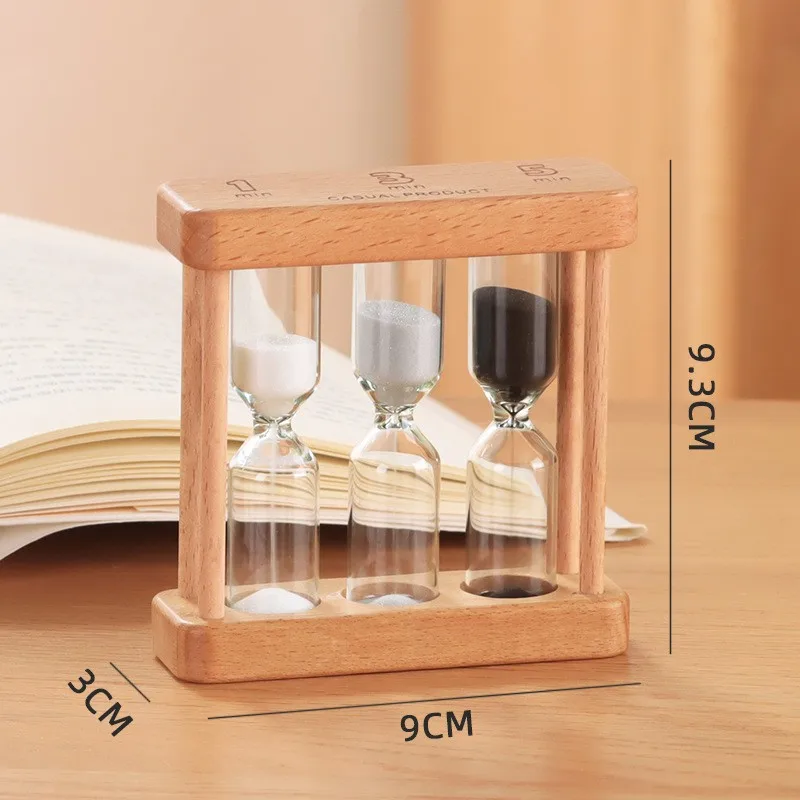The image depicts a detailed product listing or advertisement for a wooden sand timer set, likely intended for retail platforms like Walmart or Amazon. The set comprises three individual hourglasses integrated into a compact, elegant wooden frame, each with varying sand colors. From left to right, the hourglasses feature white sand, silver sand, and black sand, offering timers for one minute, three minutes, and five minutes, respectively. The inscription "casual product" is engraved on top of the frame. The overall dimensions of the hourglass set are 3 cm thick, 9 cm tall, and 9.3 cm wide. The scene is set on a light wooden table, with an open book with visible writing positioned directly behind the hourglass. The background features a mix of light brown and tan hues, maintaining an indoor, cozy atmosphere.